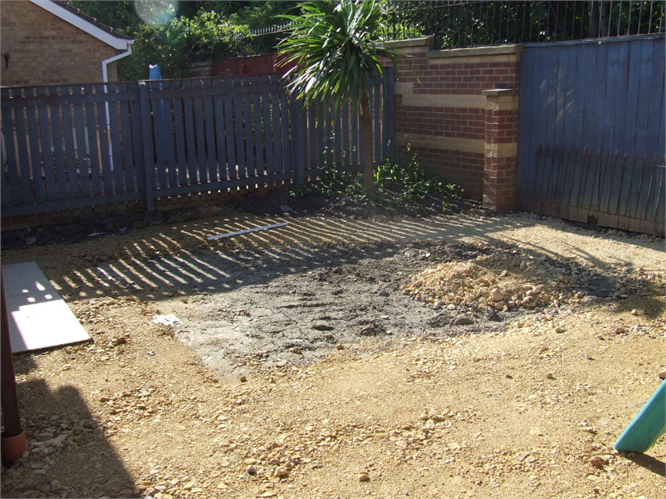In the image, a brown dirt yard occupies much of the foreground, with a depression filled with greyish dirt at its center. To the left, white square panels are arranged on the ground. The yard is bordered at the back by a blue picket fence, with additional blue fencing extending to the right, attached to a red brick wall that features a light brown brick lining interspersed. A grey stone slab sits atop this wall, supporting a metal post or the metal framework for a fence. Beyond the blue fence, lush greenery can be seen. On the left side of the image, a brown brick house with white siding climbing up to the rooftop stands prominently. Greenery also peeks over the red brick wall. In the bottom right corner, there is a patch of powdery green color, and to the left, a brick wall with an orange base is partially visible.